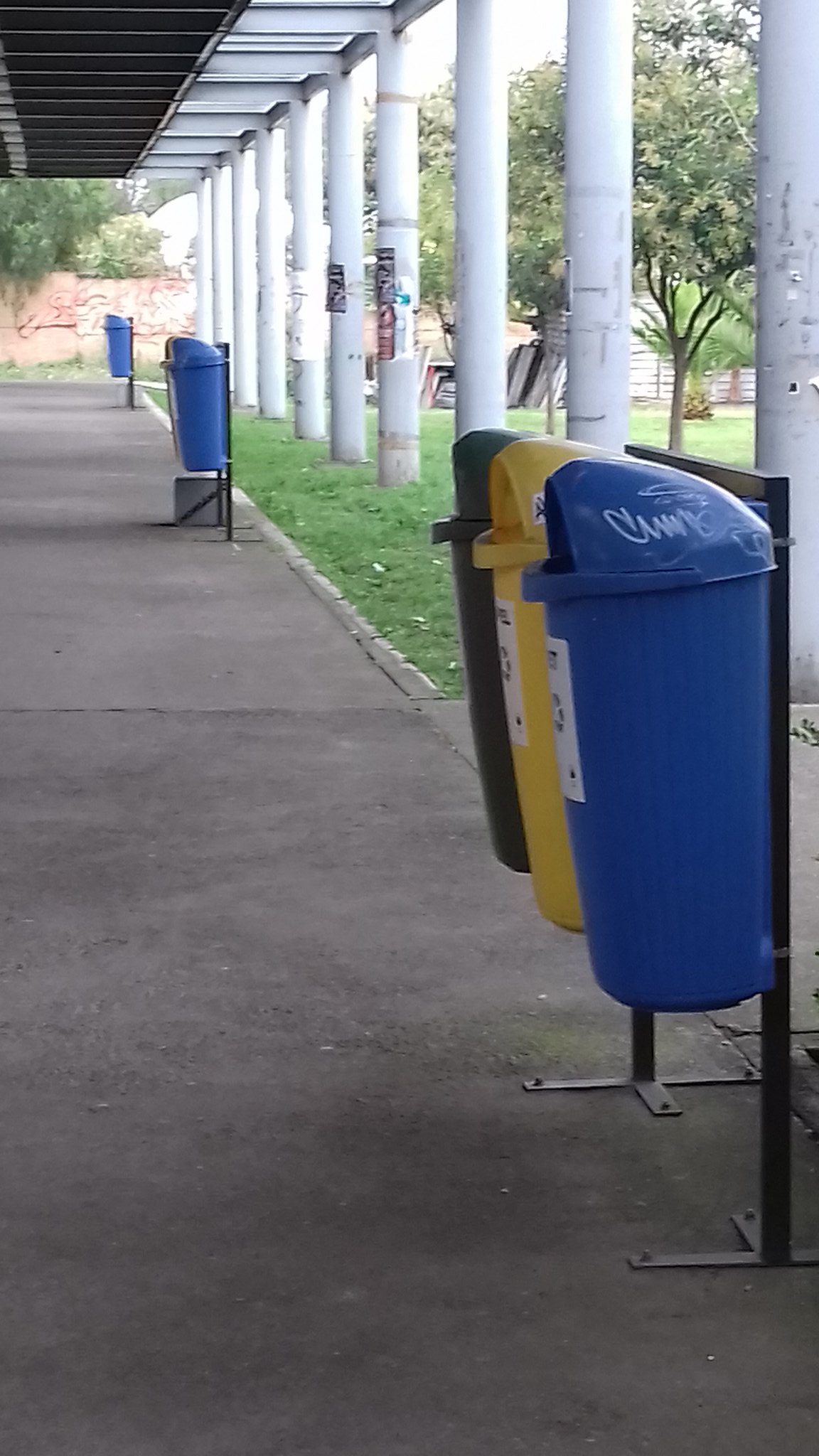The photograph captures an outdoor scene, possibly at a university campus, dominated by a dark gray cement walkway. Prominently featured on the right side are robust round stone pillars arranged closely together, supporting a structure with a brown and white overhang. This structure stretches across the view, with the roof visible in the top left corner of the image. Attached to one of the posts near the foreground is a black metal frame suspending three trash cans—blue, yellow, and black, each affixed with a white label. The blue trash can, closest to the camera, bears white marker graffiti on its lid. As the perspective recedes toward the vanishing point in the top left, additional similar frames with trash cans are seen, though from the angle only the blue cans are visible. Trees with slender trunks and yellow blooms are in the background, while a beige tall fence and a brick wall adorned with graffiti extend outward. The scene includes further details like posters on some of the pillars and objects resembling coolers or stacks of materials scattered across the grass, framed by a backdrop of tall trees.